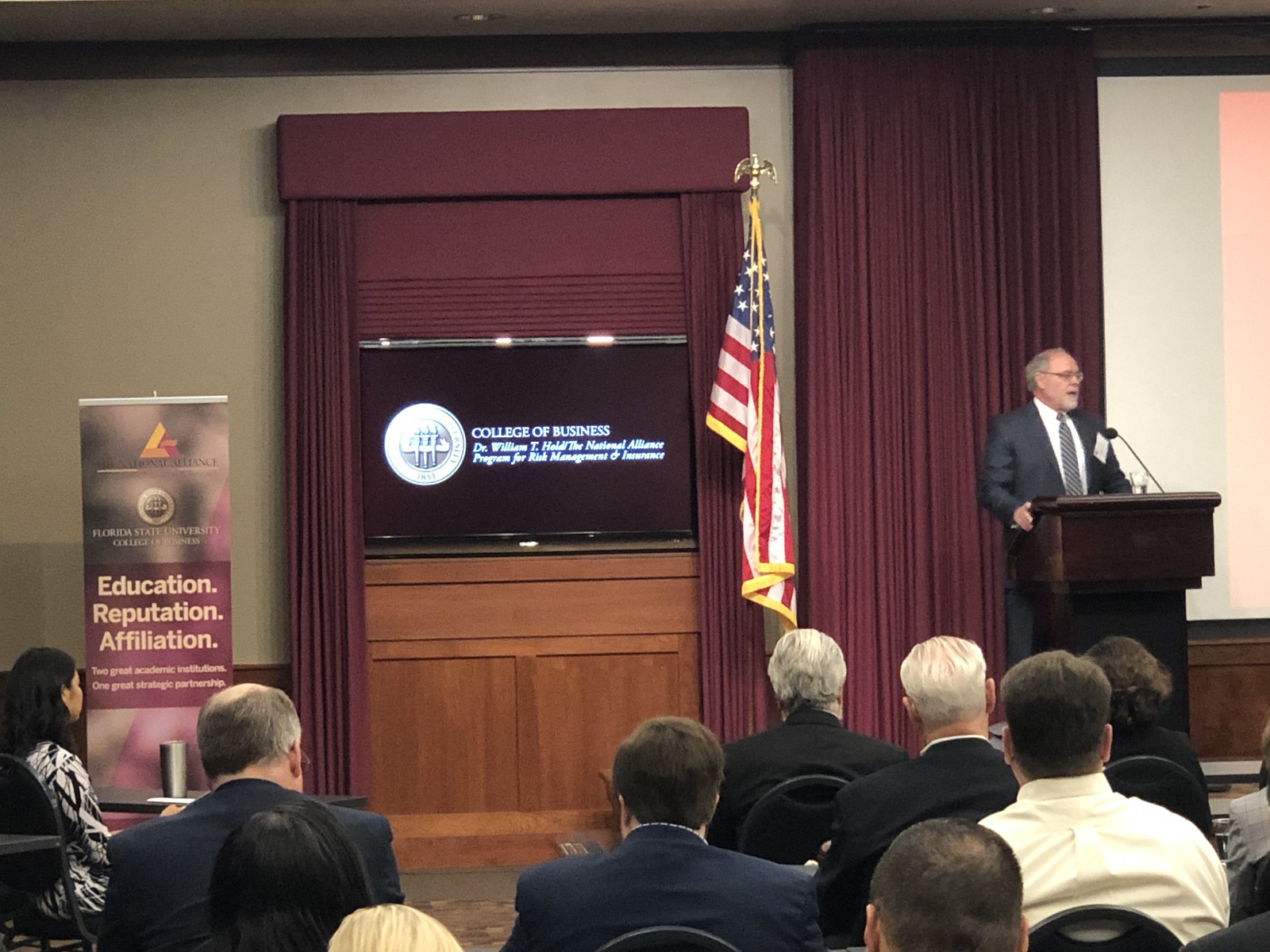The image depicts a rectangular photograph of a convention or seminar. At the forefront, a white gentleman with gray hair, glasses, and a trimmed beard stands at a dark wooden podium, speaking into a black microphone. He is dressed in a gray suit with a striped tie and a white shirt, and he appears to have a name tag on his left chest. A glass of water sits on the podium. Behind him, maroon-colored curtains frame the area, with a section closed directly behind him and another section opened to reveal a large screen. To his left stands an American flag on a pole. The screen displays the text "College of Business" and the name "Dr. William T," possibly the speaker's name. Adjacent to the screen is a tall sign that reads, "Education, Reputation, Affiliation." The audience, composed of men and women in suits and ties, sits attentively in black chairs, listening to the speaker. The scene conveys a formal, educational atmosphere dedicated to higher learning and professional development.